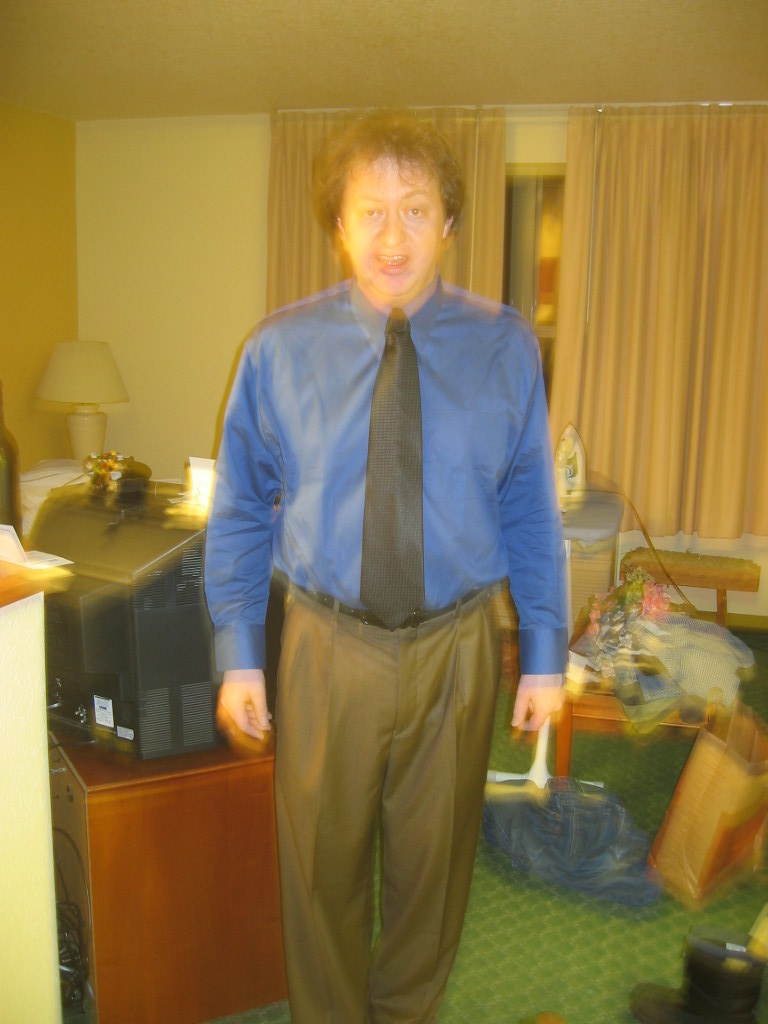In the slightly blurry photograph, a young man stands in what appears to be a somewhat impersonal hotel room. The tan walls and gold accent wall to the left, along with the tan ceiling, contribute to this impression. Heavy drapes in a dark tan color cover most of a window, revealing just a sliver of the night outside, presumably illuminated by an external light source. A small desk occupies the left-hand corner, featuring a lamp and an indiscernible object. Additionally, a blue ironing board with an iron on it is visible nearby. A brown table holds an older model television with a bulky backside, standing on a medium green carpet, which contrasts with the rest of the room’s muted colors. 

The young man in the foreground wears slightly baggy brownish pants paired with a long-sleeved, button-down collared shirt and a black tie. His curly brown hair frames his white skin, and he stares directly into the camera with his hands resting by his sides. His mouth is slightly open, giving him an expression that suggests surprise or confusion.